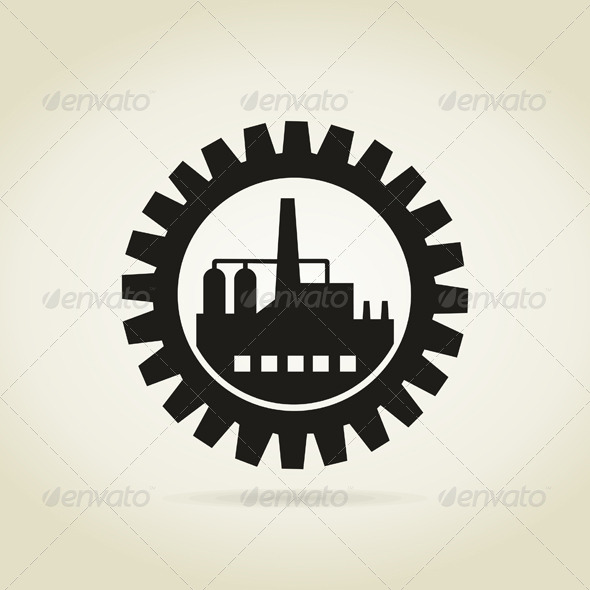The image features a square logo on a beige background with a repeated grid of light gray watermarks, arranged in three rows of three, that read "Envato." The centerpiece of the logo is a thick, dark black gear with teeth resembling those of a gear wheel. Inside this gear is a simple, black, stamped-like rendering of a factory building. The factory includes a large smokestack or chimney, two container-like structures possibly representing holds or gas tanks, and five small windows. The black ink design is set against the cream background, which can be seen through the windows of the factory illustration.